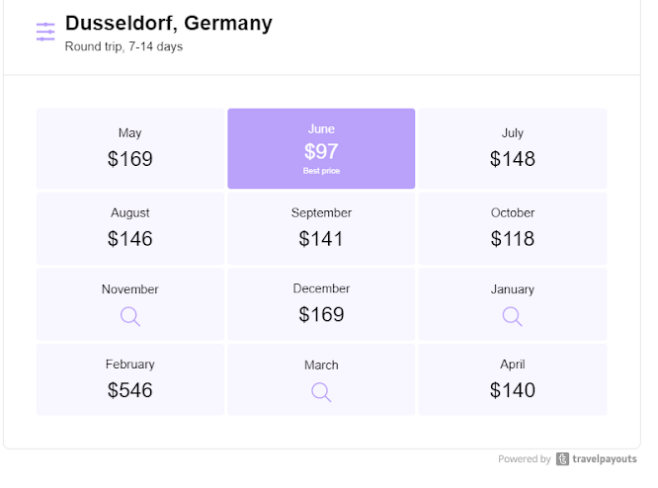The image depicts a trip booking website with a predominantly white background. In the top left corner, there is a violet-colored filter icon. To the right of the icon, bold black text reads: "Dusseldorf, Germany. Round trip 7 to 14 days." Directly below this, there is a section with light violet-colored boxes arranged in a grid—three columns wide and four rows deep. Each box contains dates and corresponding prices for trips spanning from May to April. Specifically, the prices are as follows: May - $169, June - $97, July - $148, August - $146, September - $141, October - $118, November - blank, December - $169, January - blank, February - $546, March - blank, and April - $140. The bottom right corner of the image includes the text "Powered by Travel Payouts."